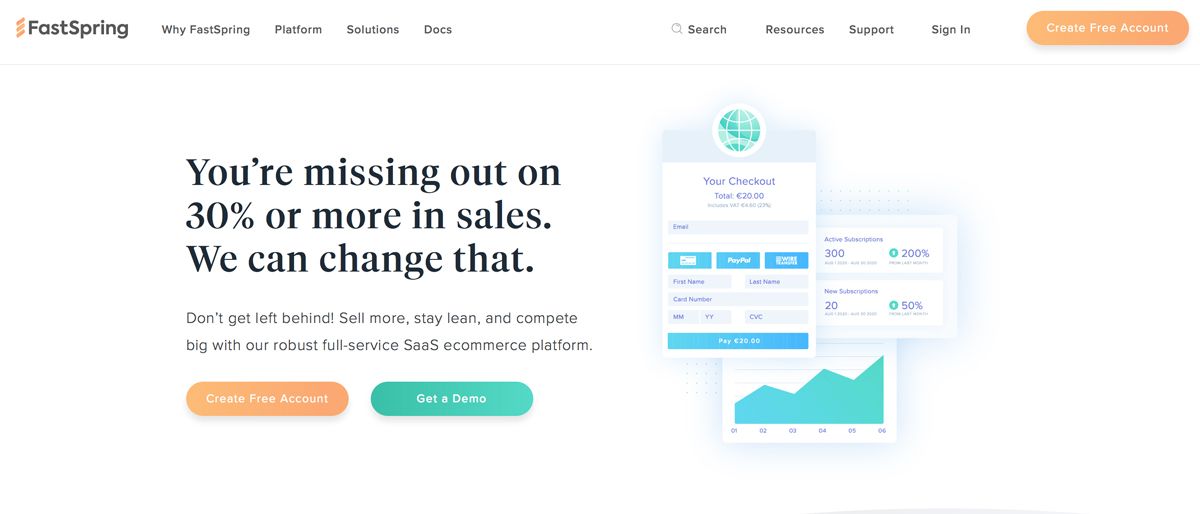**Website Caption: FastSpring Sales Introduction**

At the top of the FastSpring website, three diagonal orange lines lead to various sections: "Why FastSpring?", "Platform", "Solutions", "Docs", "Search Resources", "Support", and a "Sign In" option. There's a prominent orange button labeled "Get Free Account".

The main content area features a stark white background with bold black text stating, "You're missing out on 30% or more in sales. We can change that. Don't Get Left Behind. Sell More, Stay Lean, and Compete Big with our Robust, Full-Service SAAS eCommerce Platform."

Below this, there are two call-to-action buttons: an orange one saying "Create Free Account" and a teal one saying "Get a Demo". To the right of these buttons, there is an image of a teal and green globe at the top, which includes the text "You Are at Checkout" but the remaining text is unreadable. The image also features teal buttons. Another adjacent image depicts a teal graph starting low and progressively rising.